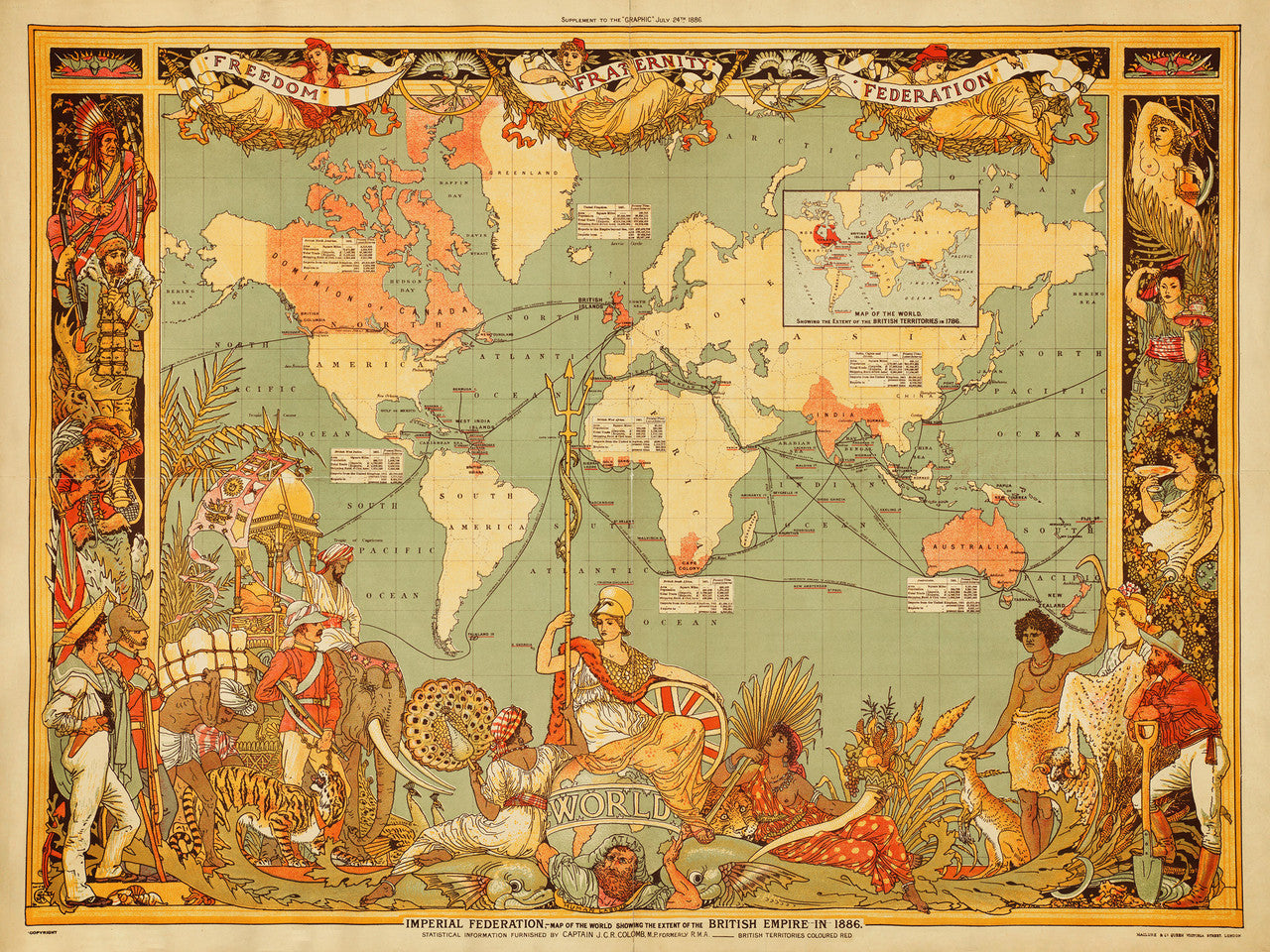This detailed image captures an ornately illustrated map of the world, titled "Imperial Federation, Map of the World, Showing the Extent of the British Empire in 1886," published by Captain J.C.R. Colonel. The map highlights the British Empire's territories in red.

Dominating the top section are three women draped in symbolic robes, each holding a banner. The woman representing "Freedom" is adorned in red and yellow, "Fraternity" is depicted in an orange or golden robe, and "Federation" in a similar orange or golden robe with a red headdress. These figures personify the core values emblazoned above the map.

Surrounding the central map, which prominently labels key regions like North America (including the Dominion of Canada and America), South America, Europe, Africa, Asia, India, and Australia, are intricate vignettes of diverse people and scenes. The text on oceans and certain areas is small but includes labels like the North Pacific Ocean, South Pacific Ocean, Atlantic Ocean, Arctic Ocean, and Alaska.

In the bottom left corner, an assortment of figures is depicted: an elephant with an Indian handler, a British soldier in a red coat and white helmet holding a rifle, a leopard or cheetah, another Indian man in traditional attire carrying a bundle, an Indian soldier, a second British soldier dressed similarly with different colored pants, a sailor with a straw hat and white pants, and finally a columned scene featuring a woman in red, a man in a blue jacket, and a Native American with a bow and arrow.

On the right side of the map, a sequence of vividly illustrated figures includes a naked woman, a woman in a green robe, a woman in a white robe, a farmer with a shovel, a woman with a straw hat, and a bare-chested Black woman petting a kangaroo. Further, a central figure of a woman, reminiscent of a Greek goddess, holds a trident while sitting atop a globe, flanked by a black woman in a red polka dot outfit and another black woman holding a peacock fan, standing barefoot. At the base, a figure identified as Atlas supports the world.

The map merges geographic detail with a diverse representation of cultures and figures, encapsulated in an elaborate Victorian artistic style reflecting 19th-century imperial attitudes and the global reach of the British Empire.